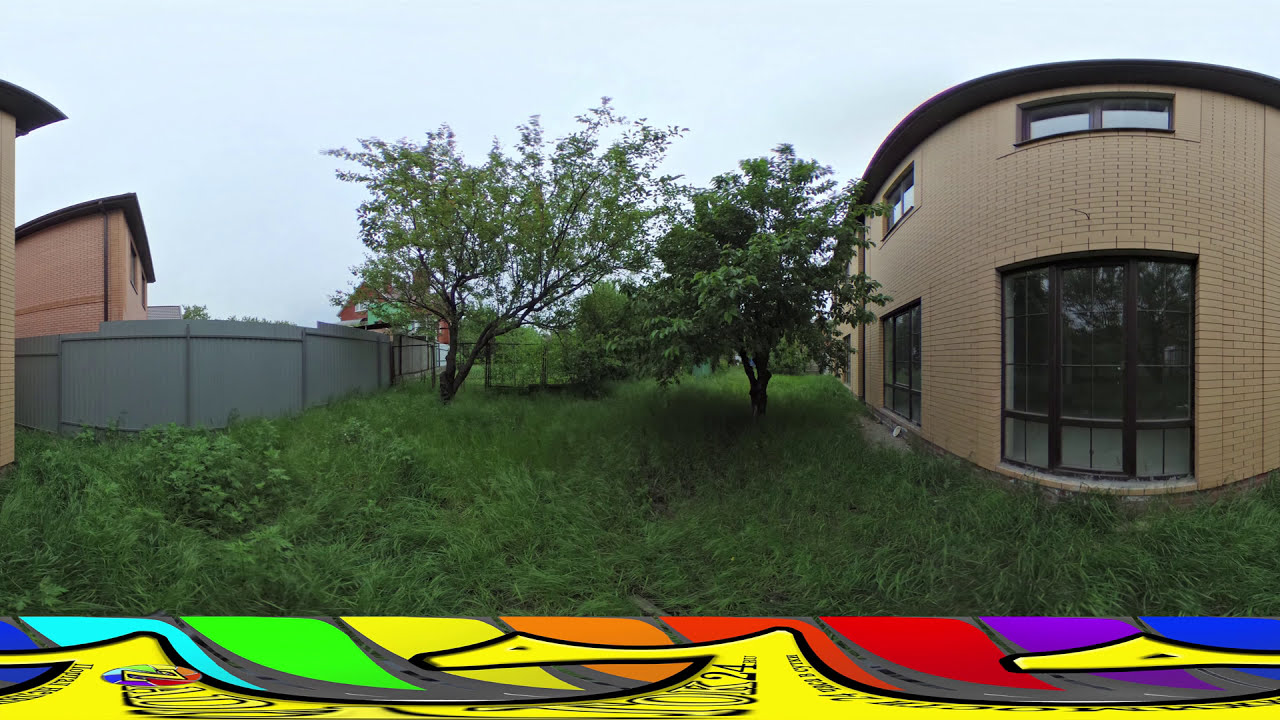The image depicts a serene backyard scene framed by a variety of elements. Dominating the lower part of the image is a vibrant graphic featuring rainbow colors interspersed with yellow and some black text reading "K-24." The backyard itself is filled with tall, lush green grass and two flourishing trees. In the center, a gray fence with a rounded design splits the scene. To the left of this fence, two taller, reddish-orange, or mauve-colored buildings with brown roofs stand behind the enclosure. On the right side is a tan brick structure with numerous large windows and a dark roof, resembling a business or residential building. Adding to the layered composition, the sky above is light blue, although somewhat hazy, giving an overcast atmosphere to the picturesque setting.